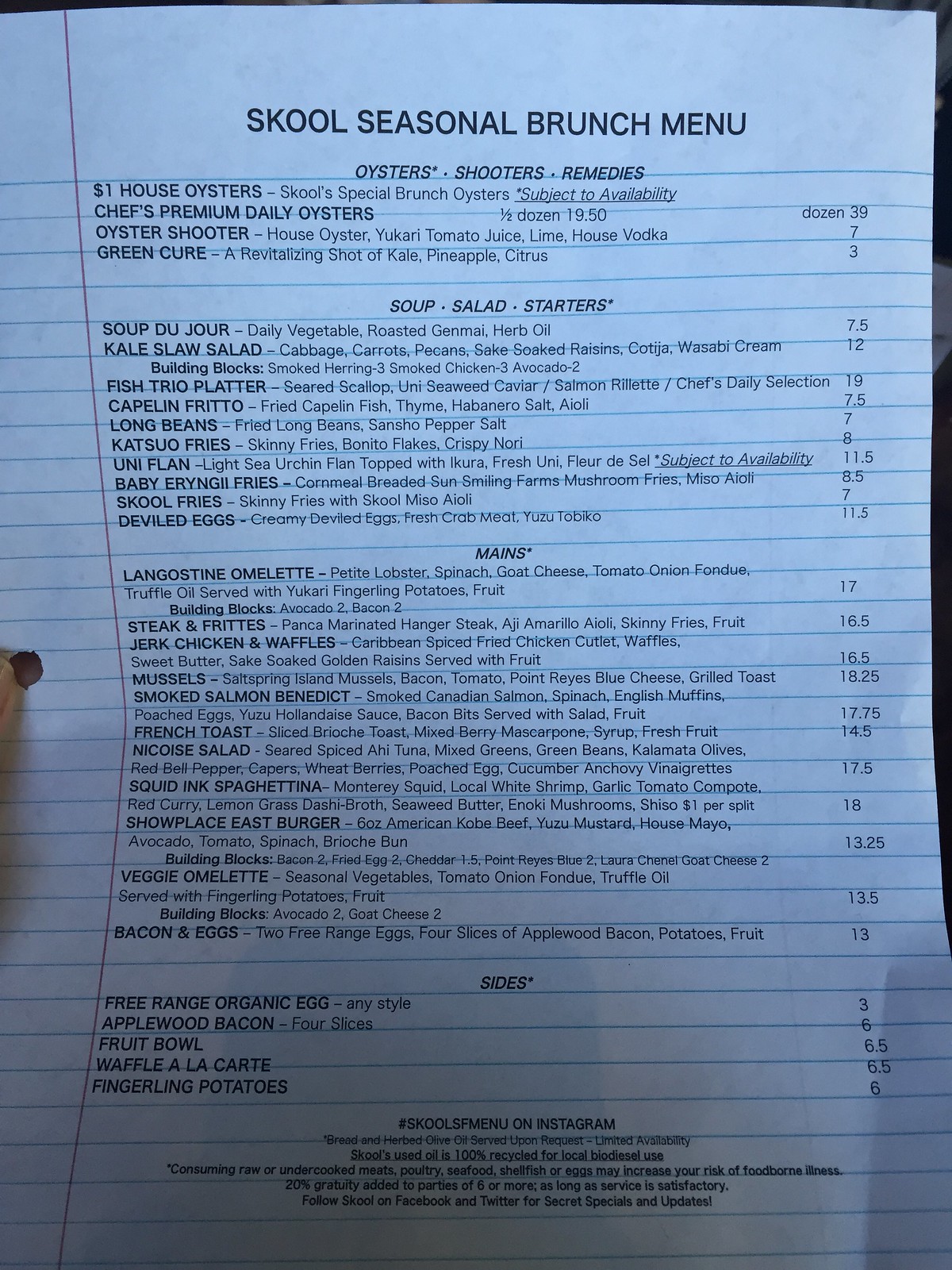**Menu Description for "SKOOL" Seasonal Brunch Menu**

**Cover Page:**
- The cover of the menu is designed like a sheet of blue lined paper with a red margin line running vertically from top to bottom on the left-hand side. Across the top of the page, the word "SKOOL" is written in a playful, child-like font, spelling out "S-K-O-O-L." Below, it is titled "Seasonal Brunch Menu."

**Oyster Shooter's Remedies:**
1. **$1 House Oysters:**
   - School Special Brunch Oysters (Subject to availability)
2. **Chef's Premium Daily Oysters:**
   - 1.5 dozen - $19.50
   - 1 each - $1.39
3. **Oyster Shooter - $7.00:**
   - Ingredients: House oyster, gnocchi, tomato juice, lime, house vodka.
4. **Green Cure - $3.00:**
   - Description: Revitalizing shot of kale, pineapple, and citrus.

**Soup Salad Starters:**
1. **Soup Du Jour - $7.50:**
   - Daily vegetable roasted genmai, herb oil.
2. **Kale Slaw Salad - $12.00:**
   - Ingredients: Cabbage, carrots, pecans, sake-soaked raisins, cotija cheese, wasabi cream.

**Building Blocks:**
1. **Smoked Herring - $3.00**
2. **Smoked Chicken - $3.00**
3. **Avocados - $2.00**
4. **Fish Trio Platter - $19.00:**
   - Features: Seared scallops, uni seaweed caviar, salmon roulette, chef's daily selection.
5. **Capelin Frito - $7.50:**
   - Ingredients: Fried capelin fish, thyme, habanero salt, aioli.
6. **Long Beans - $7.00:**
   - Description: Fried long beans, Sancho pepper salt.
7. **Katsuo Fries - $8.00:**
   - Ingredients: Skinny fries, bonito flakes, crispy nori.
8. **Uni Flan - $11.00:**
   - Description: Light sea urchin flan topped with yuzu fresh uni, fleur de sel (Subject to availability).
9. **Baby Eryngii Fries - $8.00:**
   - Description: Cornmeal breaded mushroom fries from Sun Smiling Farms, miso aioli.
10. **School Fries - $7.00:**
    - Description: Skinny fries with school miso aioli.
11. **Deviled Eggs - $11.00:**
    - Ingredients: Creamy deviled eggs, fresh crab meat, tobiko.

**Mains:**
1. **Langoustine Omelette - $17.00:**
   - Ingredients: Petite lobster, spinach, goat cheese, tomato, onion fondue, truffle oil. Served with yuki fingerling potatoes and fruits.
2. **Building Blocks:**
   - Avocado - $2.00
   - Bacon - $2.00
   - Steak Fritters - $16.50:
     - Pan-seared marinated hanger steak, aji amarillo aioli, skinny fries, fruit.
3. **Jerk Chicken Waffles - $16.50:**
   - Ingredients: Caribbean spiced fried chicken cutlets, waffles, sweet butter, sake-soaked golden raisins. Served with fruit.
4. **Mussels - $18.25:**
   - Ingredients: Salt Spring Island mussels, bacon, tomato, Point Reyes blue cheese, grilled toast.
5. **Smoked Salmon Benedict - $17.75:**
   - Ingredients: Smoked Canadian salmon, spinach, English muffins, poached eggs, yuzu hollandaise sauce, bacon bits. Served with salad and fruit.
6. **French Toast - $14.50:**
   - Ingredients: Sliced brioche toast, mixed berries, mascarpone, syrup. Served with fresh fruit.
7. **Nikko Salad - $17.50:**
   - Description: Served with spiced asahi tuna, mixed greens, green beans, calamari olives, red bell peppers, capers, wheat berries, poached egg, cucumber, anchovy vinaigrette.
8. **Squid Ink Spaghettini - $18.00:**
   - Ingredients: Monterey squid, local white shrimp, garlic tomato compote, red curry lemongrass dashi broth, seaweed butter, enoki mushrooms, seiko.
   - Split plate fee: $1.00
9. **Show Place East Burger - $13.25:**
   - Ingredients: 6oz American Kobe beef, yuzu mustard, house mayo, avocados, tomatoes, spinach, brioche bun.
   - Add-ons: Bacon, fried eggs.
10. **Veggie Omelette - $13.05:**
    - Ingredients: Seasonal vegetables, tomato, onion fondue, truffle oil. Served with fingerling potatoes.
    - Add-ons: Avocado - $2.00, goat cheese - $3.00.
11. **Bacon and Eggs - $13.00:**
    - Ingredients: 2 free-range eggs, 4 slices of applewood bacon, potato, fruit.

**Sides:**
1. **Free Range Organic Egg (Any Style) - $3.00**
2. **Applewood Bacon (4 Slices) - $6.00**
3. **Fruit Bowl - $6.50**
4. **Waffle a la Carte - $6.50**
5. **Fingerling Potatoes - $6.00**

**Note:** Additional text on the menu is written in black but is too small to read.